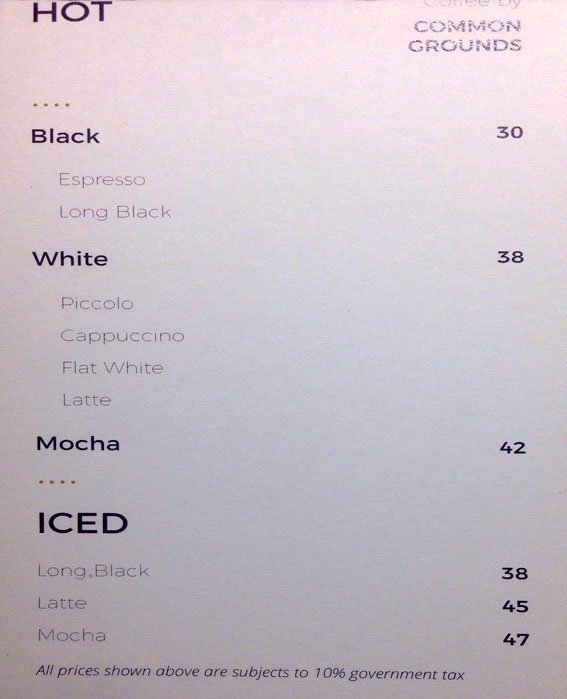This image showcases a meticulously detailed coffee menu on a predominantly white background, accented with subtle pink and blue elements. In the upper left corner, there is a bold, blue header that reads "Hot." Opposite, in the upper right corner, the name of the establishment, "Common Grounds," is presented in faded text. Below this, the menu is divided into distinct categories with corresponding prices.

The first section is titled "Black" in bold, with items listed underneath in unbolded blue text: "Espresso" and "Long Black." The price for items in this category is listed as $30 to the right. Following this, another bold header reads "White," priced at $38. Under this category, the items "Piccolo," "Cappuccino," "Flat White," and "Latte" are listed in the same unbolded blue text. The next item, "Mocha," stands alone without subcategories, priced at $42.

Further down, the menu introduces a section for "Iced" beverages, indicated by a larger bolded header. This section includes "Long Black" at $38, "Latte" at $45, and "Mocha" at $47. A note at the bottom of the menu mentions that "All prices shown above are subject to 10% government tax," ensuring clarity for potential customers.